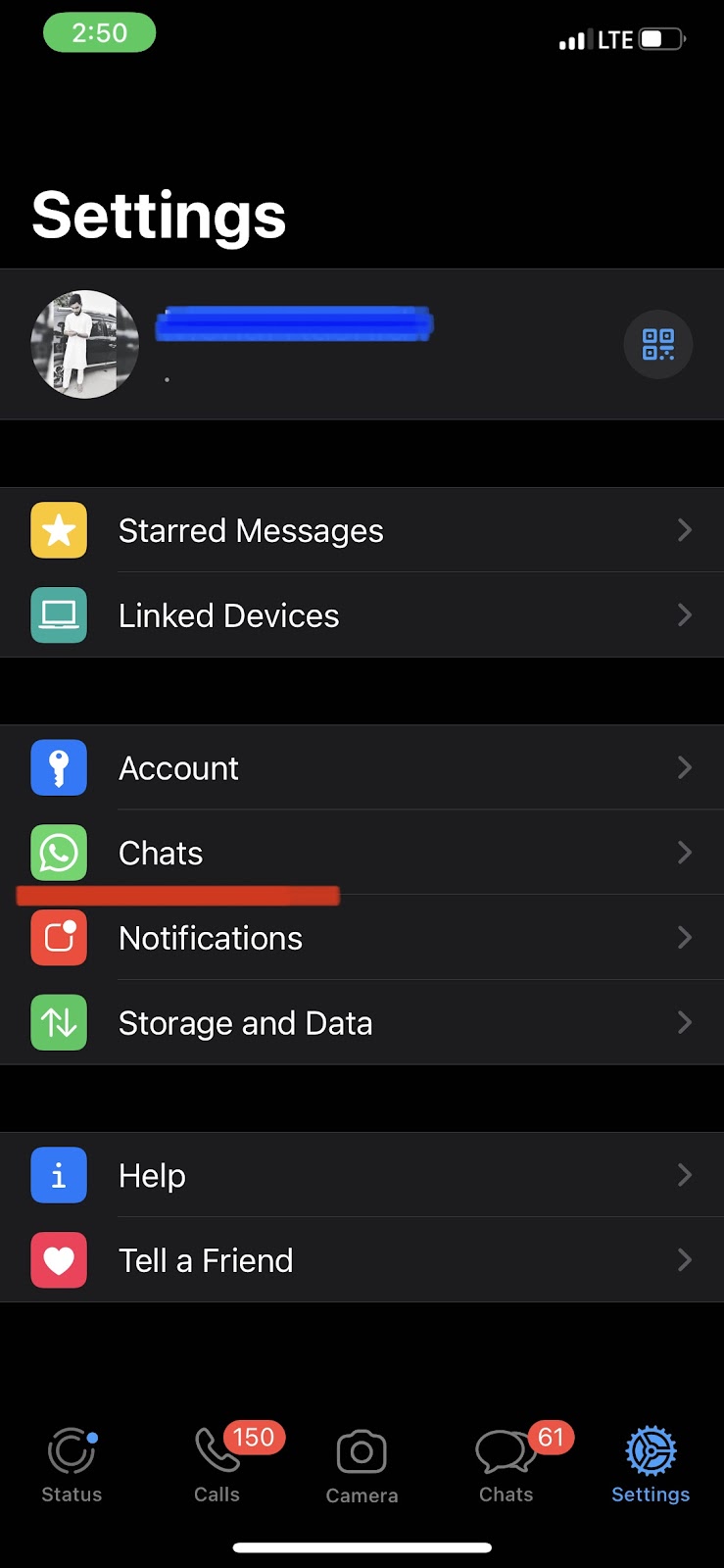Screenshot of a smartphone displaying the settings menu. The background is a combination of black and very dark gray, with the word "Settings" in white at the top. Below the title, there's a black-and-white icon photo of a person, dressed in white and looking down at their phone. Next to the photo, the person's name is obscured by a blue marking.

Underneath the profile section, a list of menu items is displayed:

1. **Starred Messages**: Represented by a yellow box with a white star inside.
2. **Linked Devices**: Identified by a turquoise square containing a white computer icon.
3. **Account**: Symbolized by a blue square with a white key.
4. **Chats**: Marked by a green square with a white telephone inside a message icon.
5. **Notifications**: Illustrated by a red square with a white bell inside a small circle.
6. **Storage and Data**: Depicted by a green square with two white arrows.
7. **Help**: Shown as a blue square with a lowercase white "i".
8. **Tell a Friend**: Indicated by a red square with a white heart inside.

At the bottom of the screen, several icons relevant to phone functions are displayed:

- **Status**: An icon labeled "Status."
- **Calls**: Indicated with a red oval containing the number 150, representing missed or recent calls.
- **Camera**: Represented by a standard camera icon.
- **Chats**: Displayed with a red oval showcasing the number 61, indicating unread messages.
- **Settings**: Marked with a blue settings icon.